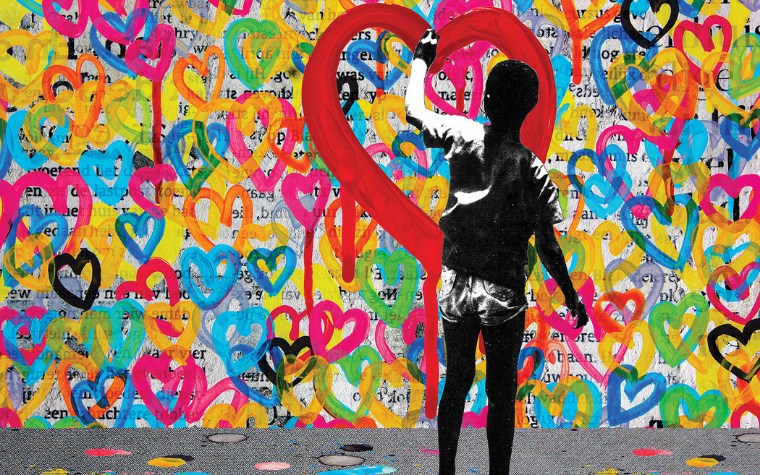This rectangular, horizontal artwork depicts a young man in black and white, wearing shorts and a short-sleeved t-shirt, with close-cropped hair. He stands in the right center of the image, his right arm down by his side and his left arm raised as if he's painting. The background features a wall covered with enlarged newsprint text obscured by numerous multicolored hearts in shades of pink, blue, green, orange, yellow, and black. The text on the wall is in a serif font, but it's largely unreadable due to its small size and the overlay of hearts. The focal point is a large red heart the young man appears to be painting with his left hand. Scattered paint splatters in pink, yellow, gray, and blue are visible on the dark gray ground beneath him, adding to the vibrant and dynamic feel of the scene.